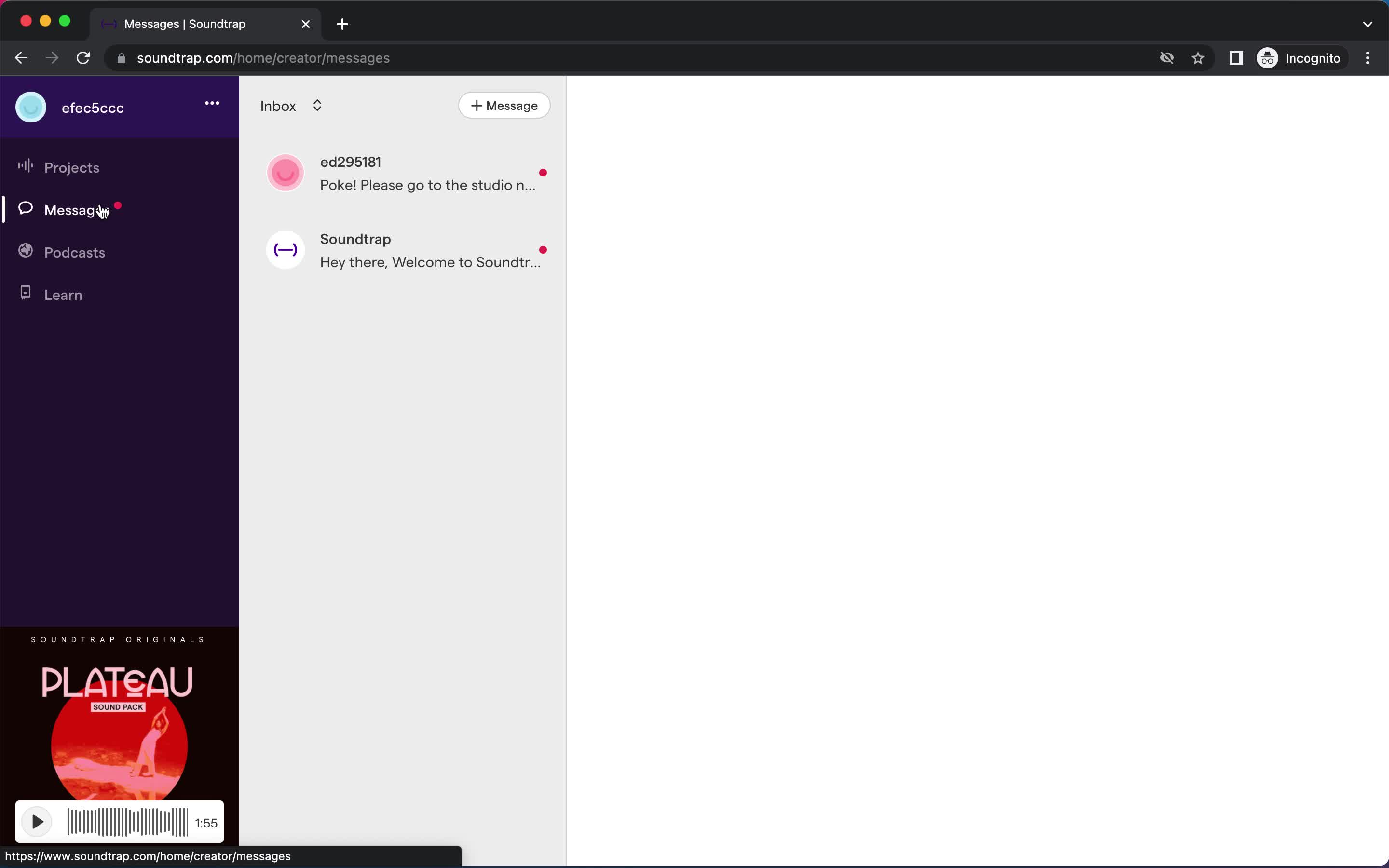The image displays a webpage from the website "soundtrap.com" at the URL path "home/creator/messages." On the left side of the page, a menu with a purple background is visible, featuring various buttons or tabs. The user profile displayed has the ID "E-F-E-C-5-C-C-C." Under the username, several menu options are listed, including "Projects," "Messaging," "Podcast," and "Learn."

At the bottom left side of the screen, an advertisement for an album is featured, reading "Soundtrap Originals: Pilatiawu Soundtrack." There is a pink circular play button beneath the ad, indicating that the soundtrack has a duration of 1 minute and 55 seconds.

On the right side of the screen, there is an inbox section with a grey background. The inbox contains two messages. The first message is from the user "ED295181," stating "POG, please go to the studio," and it has a pink dot next to it, signifying that the message is unread. The second message is from "Soundtrap," welcoming the user with "Hey there, welcome to Soundtrap," also marked with a pink dot to indicate it is unread.